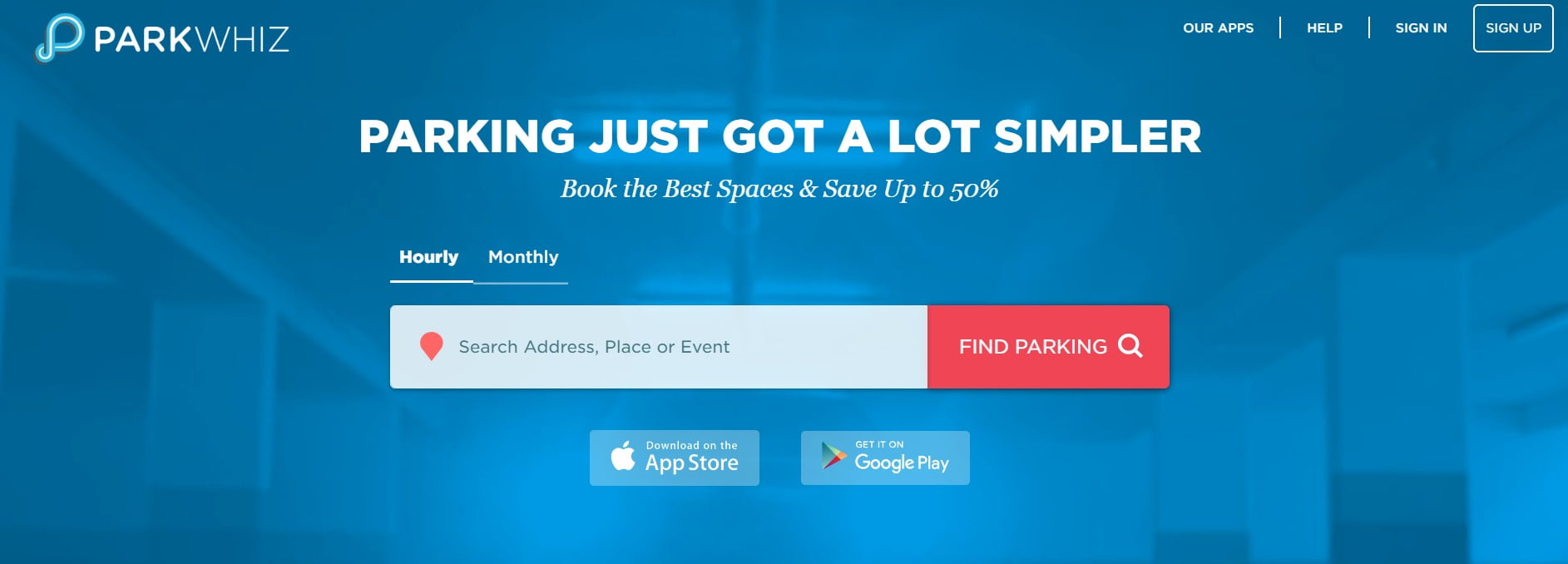The image displays the first page of ParkWiz. The logo, situated to the left of the word "ParkWiz," features a stylized number 8, with one of the circles being much smaller, designed to convey an infinite loop, positioned diagonally. The word "ParkWiz" is split into two styles: "Park" is bold and white, while "Wiz" is in thinner white text, all set against a blue background. The tagline "Parking just got a lot simpler. Book the best spaces and save up to 50%," prominently stands out.

Below the tagline, there is a search bar with the placeholder text "Search address, place or event." The search button next to it is red. Users can choose to search for parking spaces either by hourly or monthly options. Beneath the search bar, there are prompts to download the app from the App Store or Google Play.

In the upper right corner of the page, there are options labeled "Our Apps," "Help," "Sign In," and "Sign Up."